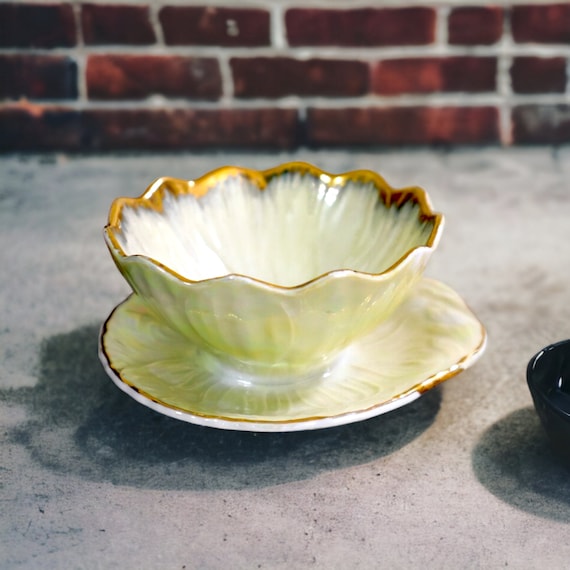The image depicts a delicate teacup or bowl with a shape reminiscent of a tulip, featuring wide, scalloped edges painted in gold. The exterior of both the bowl and its matching saucer is a near-white, cream color with wavy striations and a textured finish. Both items are accented by thin, golden edges, adding to their elegant appearance. These pieces rest on a gray, stone or cement surface, casting a dark gray shadow beneath them. To the bottom right, there's a smaller, glossy black bowl. The scene is set against a dark red brick wall, which serves as the background, enhancing the contrast and highlighting the intricate details of the teacup and saucer.